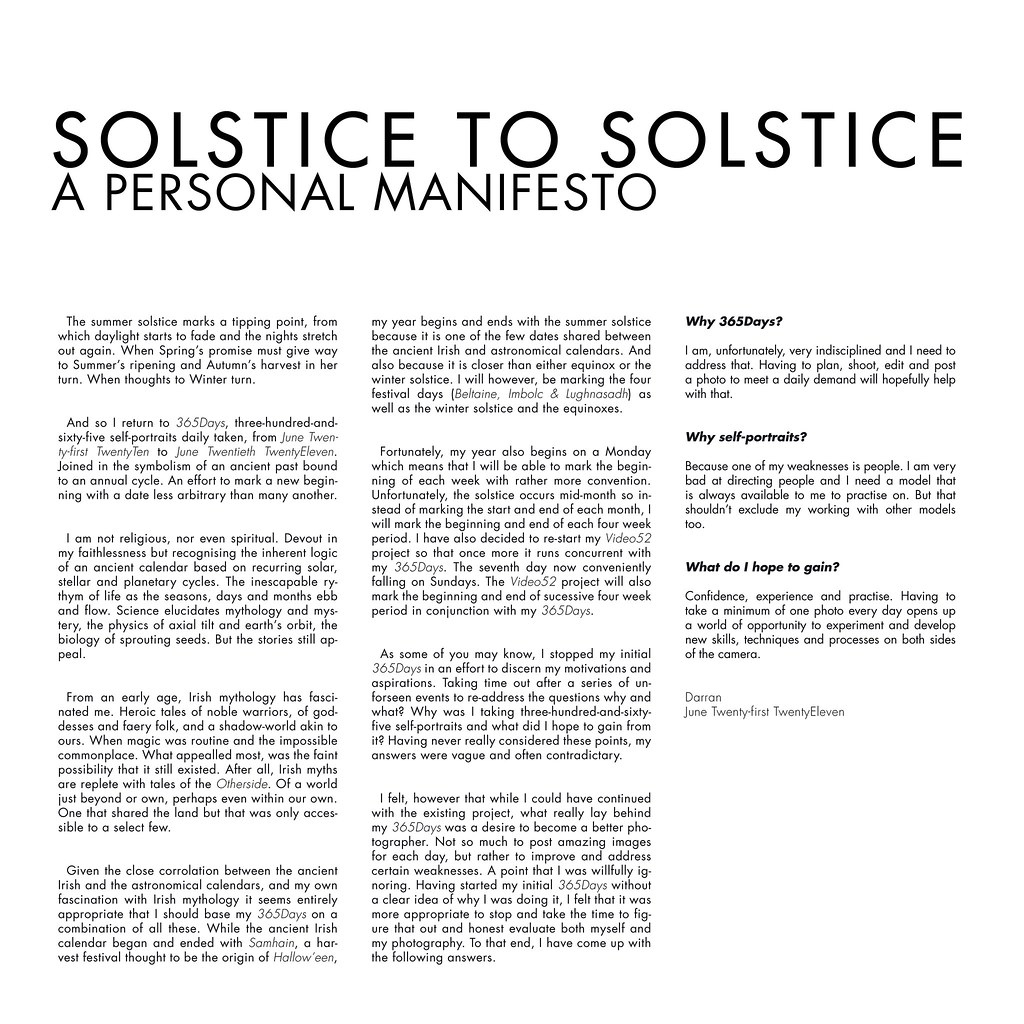The image features a text-based document titled "Solstice to Solstice, A Personal Manifesto," displayed on a white background in black font. The title at the top is in a larger font, while the remaining text is arranged in three columns in a smaller font, resembling a newspaper article. The first column begins with two paragraphs explaining the significance of the summer solstice as a turning point in the annual cycle, marking the start of a 365-day journey of daily self-portraits from June 21st, 2010, to June 20th, 2011. The text connects this project to ancient traditions and emphasizes its role in heralding a meaningful new beginning. The second column has a merged paragraph from the first and delves into more narrative detail. The third column contains bold headings for sections such as "Why 365 days?", "Why self-portraits?" and "What do I hope to gain?", each followed by explanatory paragraphs. The section "Why 365 days?" reveals the author's struggle with discipline and the daily commitment intended to address this issue. The document is signed "Darren, June 21st, 2011," with the date spelled out in words.